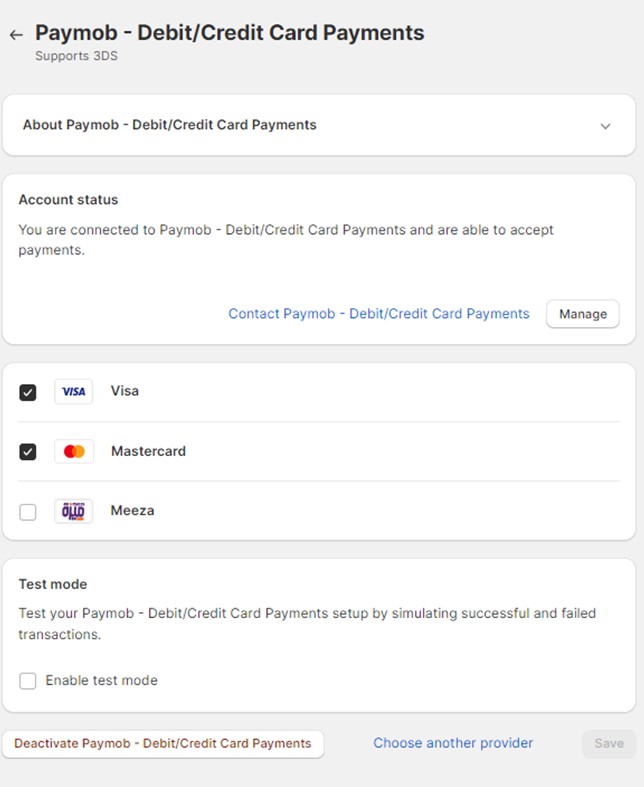**Detailed Caption:**
The image depicts a vertical interface screen from a computer or smart device showcasing a payment option. The background is a light to medium gray. At the top of the screen, there is a left-pointing arrow. On the left-hand side, text appears in black stating "PayMob - Debit/Credit Card Payments" with a subtext underneath that mentions "Supports 3D Secure (3DS)".

Below this, a white rounded-rectangle box features black text saying "About PayMob - Debit/Credit Card Payments" with a right-pointing arrow indicating an option to expand for more information.

Following that, a slightly larger rounded-rectangle box is titled "Account Status" in bold black text. Underneath in lighter text, it reads "You are connected to PayMob - Debit/Credit Card Payments and are able to accept payments". At the bottom of this section, blue text states "Contact PayMob - Debit/Credit Card Payments" and a smaller box labeled "Manage" is also visible.

The next segment of the interface is a box divided into three parts: one part includes a checkmark and the Visa logo, another part a checkmark and the MasterCard logo, and the final part has an unchecked icon for Maestro, each respective to their brand's distinctive iconography.

At the bottom, another white box includes instructions for "Test Mode" where users can simulate successful and failed transactions to test their PayMob - Debit/Credit Card Payments setup. The text indicates options to "Enable Test Mode", "Deactivate PayMob", "Choose Another Provider" as well as a "Save" button, which is currently not illuminated.